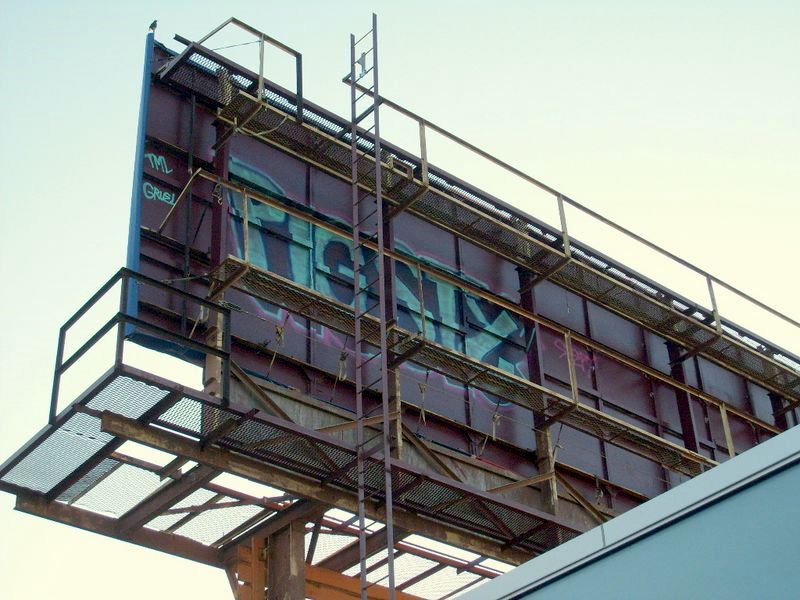The image captures the back view of a billboard on a slightly cloudy day with a light blue sky. The billboard structure features three horizontal walkways, almost like narrow bridges, which are likely used by workers for maintenance. These walkways are secured with guard rails for safety. The front of the billboard is a large rectangular surface supported by an intricate framework of vertical, horizontal, and X-shaped metal reinforcements, particularly strengthened at the bottom. A ladder is visible on the left side, extending from below the billboard to above it. Additionally, an orange beam is noticeable beneath the billboard, partially obscured but extending from under the structure. Below this, a blue wall adds another layer of color and complexity to the scene.